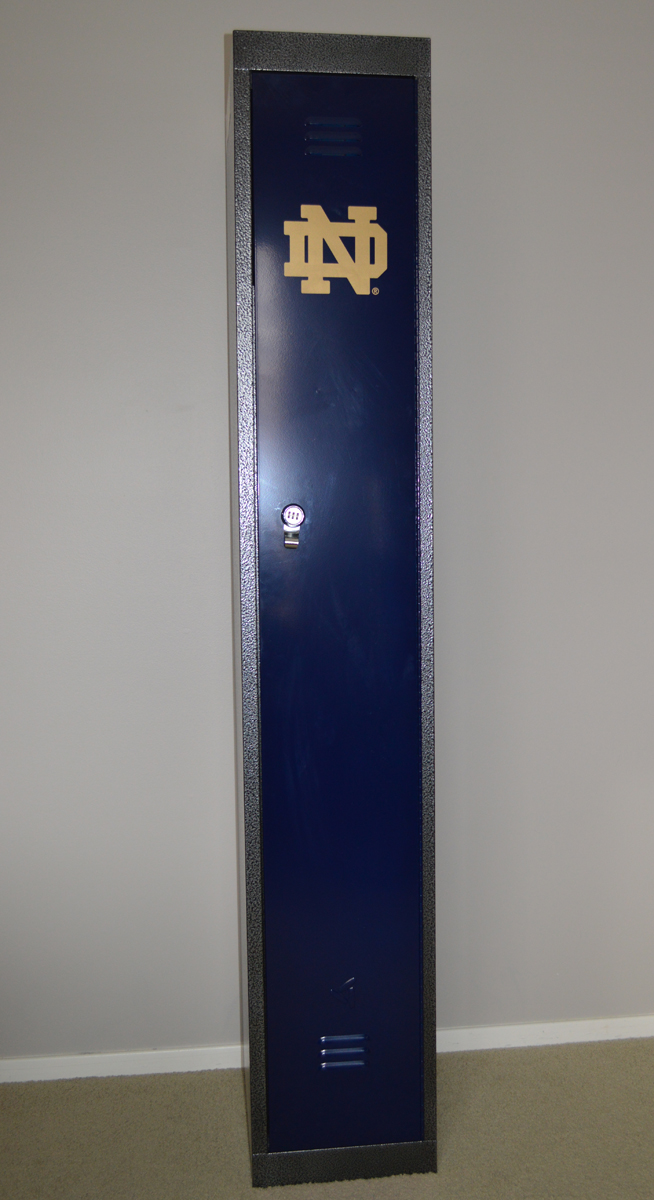The image depicts a tall, rectangular locker standing against a white wall with a grayish carpeted floor. The locker is primarily metallic silver with a front door painted in a dark navy blue. This door features the gold Notre Dame logo at the top, consisting of an interlocking 'N' and 'D'. The logo includes a trademark symbol. The locker is unique in that it stands alone rather than as part of a row of lockers. There is a silver lever handle on the door, designed to open the locker. Below, there are ventilation ports near the bottom, and a small, tilted triangular logo, likely the manufacturer's mark, can be seen just above these ports. The setting appears to be a personal space, possibly in someone's home or office, hinting at the owner's connection to or admiration for Notre Dame. The light source is positioned behind the camera, illuminating the scene evenly.